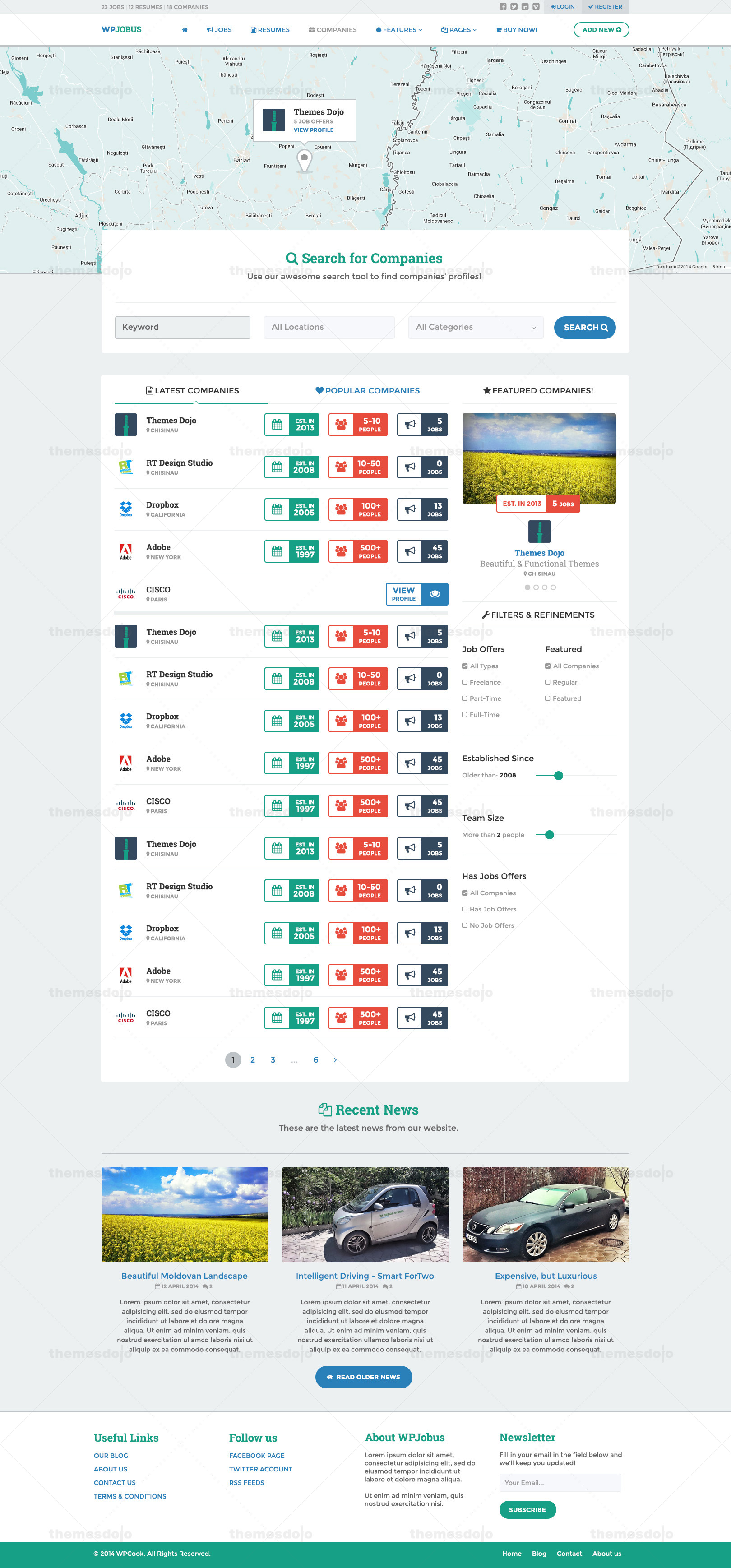The image presented is a vertically elongated screenshot of a website, capturing an extensive view of the page content, though much of the text is too small to read. At the very top, there is a horizontally rectangular map, providing a visual focal point. Below the map, the background of the frame is predominantly gray. An overlaid white search box invites users to "Search for companies," situated above a vertical listing of what appear to be various companies, all enclosed within a vertically rectangular white box. Towards the bottom of the frame, a section labeled "Recent News" is visible, displaying three images side by side, each accompanied by unreadable titles and descriptions of the respective stories. The website or application's identity remains unclear due to the indistinct detail of the text and icons throughout the screenshot.